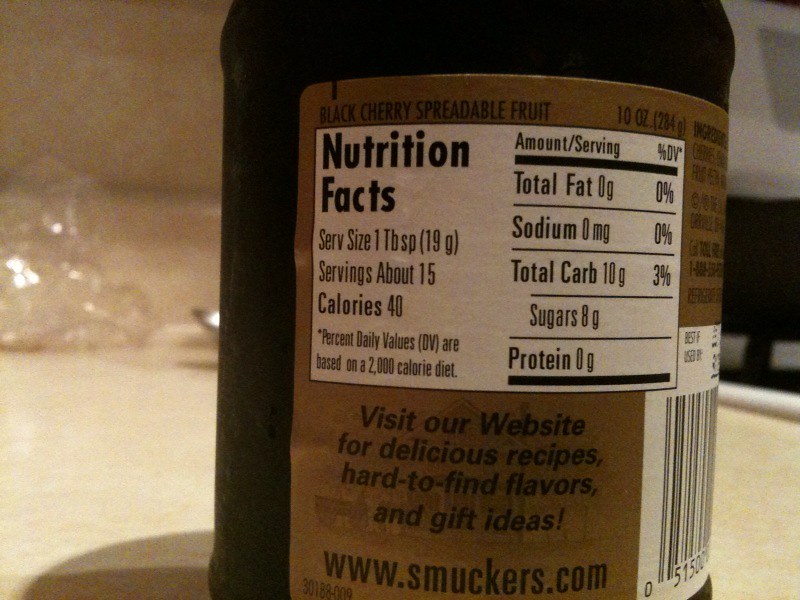This image showcases the nutrition facts label on the back of a jar of Smucker's Black Cherry Spreadable Fruit. Upon closer inspection, one can see the distinctive brown label adorned with white text for clear visibility. Information encircles the jar, including nutritional details and a UPC barcode. The label encourages customers to visit their website for delicious recipes, hard-to-find flavors, and unique gift ideas.

The nutritional facts specify that each serving size is 1 tablespoon, with approximately 15 servings per container. Each serving contains 40 calories, 0 grams of total fat, 0 milligrams of sodium, 10 grams of total carbohydrates, 8 grams of sugars, and 0 grams of protein, making it a flavorful yet low-calorie spread option.